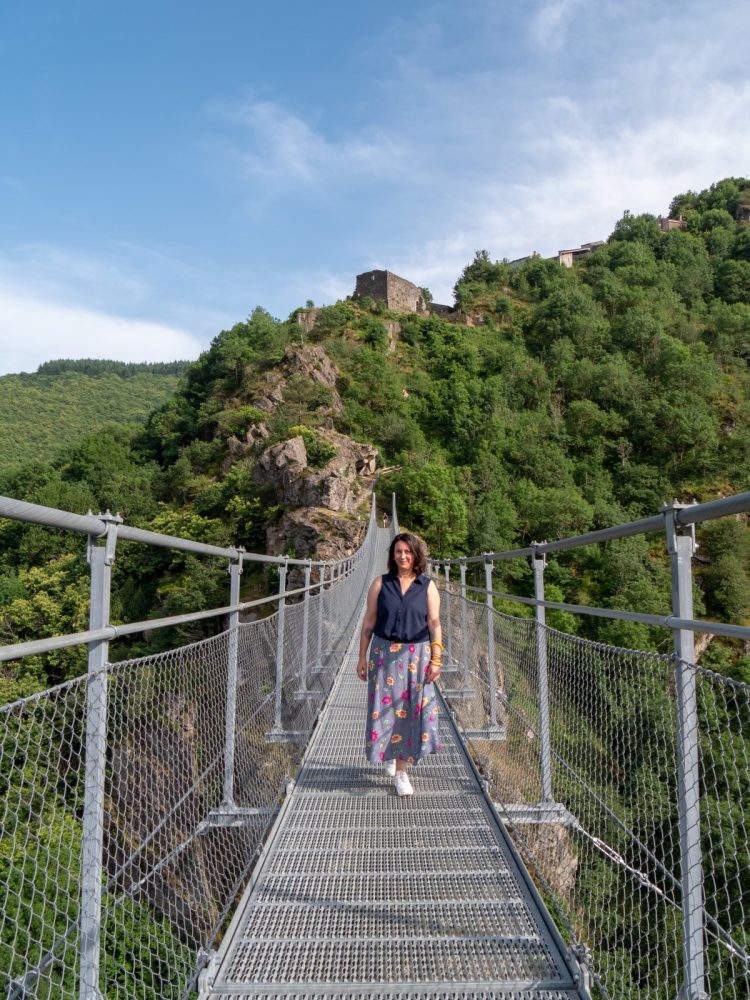In this photograph, a woman is walking across a long metal pedestrian bridge that spans a wide canyon, connecting one forested cliff to another. The viewpoint is straight down the bridge, allowing a clear view of its metal handrails and protective fencing. The woman, with light skin and brown hair, is centrally positioned in the frame, walking towards the viewer. She is dressed in a dark blue blouse, a light blue long skirt adorned with red and yellow flowers, and white walking shoes. Although she appears to be alone on the bridge, there is a faint, indistinct figure in the background. The bridge leads into a rocky cliff on the opposite side, surrounded by dense trees. The scene captures a mostly sunny day with few clouds dotting the sky, and the environment is vividly green with lush trees and rugged terrain flanking the bridge. The overall setting is tranquil, emphasizing the outdoor connection between the two large hills or mountains.